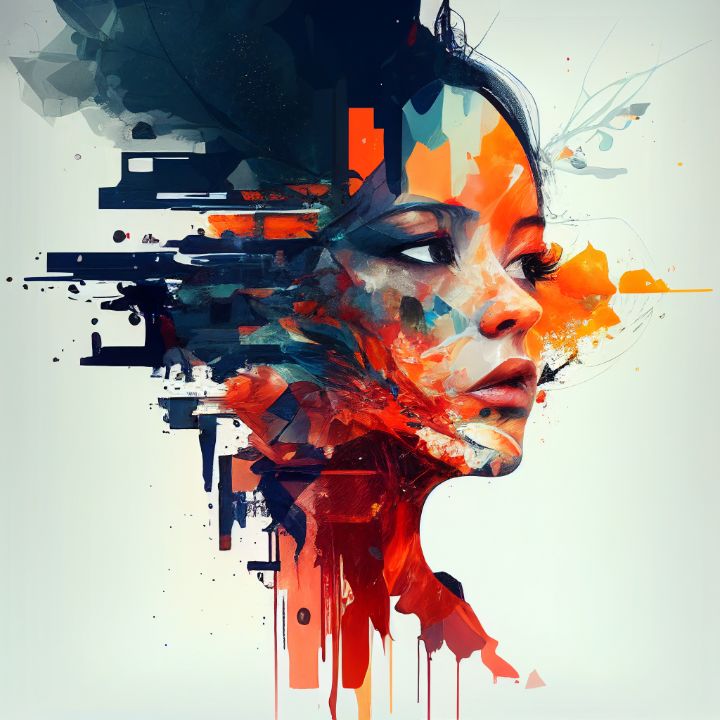This is a piece of digital modern art featuring a woman's face diagonally oriented toward the viewer but looking to the right side of the image. Her facial features are distinct, with long eyelashes, brown eyes, and pink lips. She has fair, skin-colored peach tones accented by dramatic splashes of color. A notable red splatter on her cheek smears downward into her neck, mingling with other shades like orange, teal, green, dark teal, and blue. Her black hair, styled in a voluminous, almost beehive fashion, is layered with graffiti-style silhouettes resembling a city skyline, tilted to the left. These fragmented building shapes transition into smoke-like forms at the top of the image. The background is predominantly a flat, tan color, which frames the detailed coloration and textured splatters that extend outward from her face and the rest of her head. The overall effect is a blend of realistic facial features and abstract, splattered artistic elements.